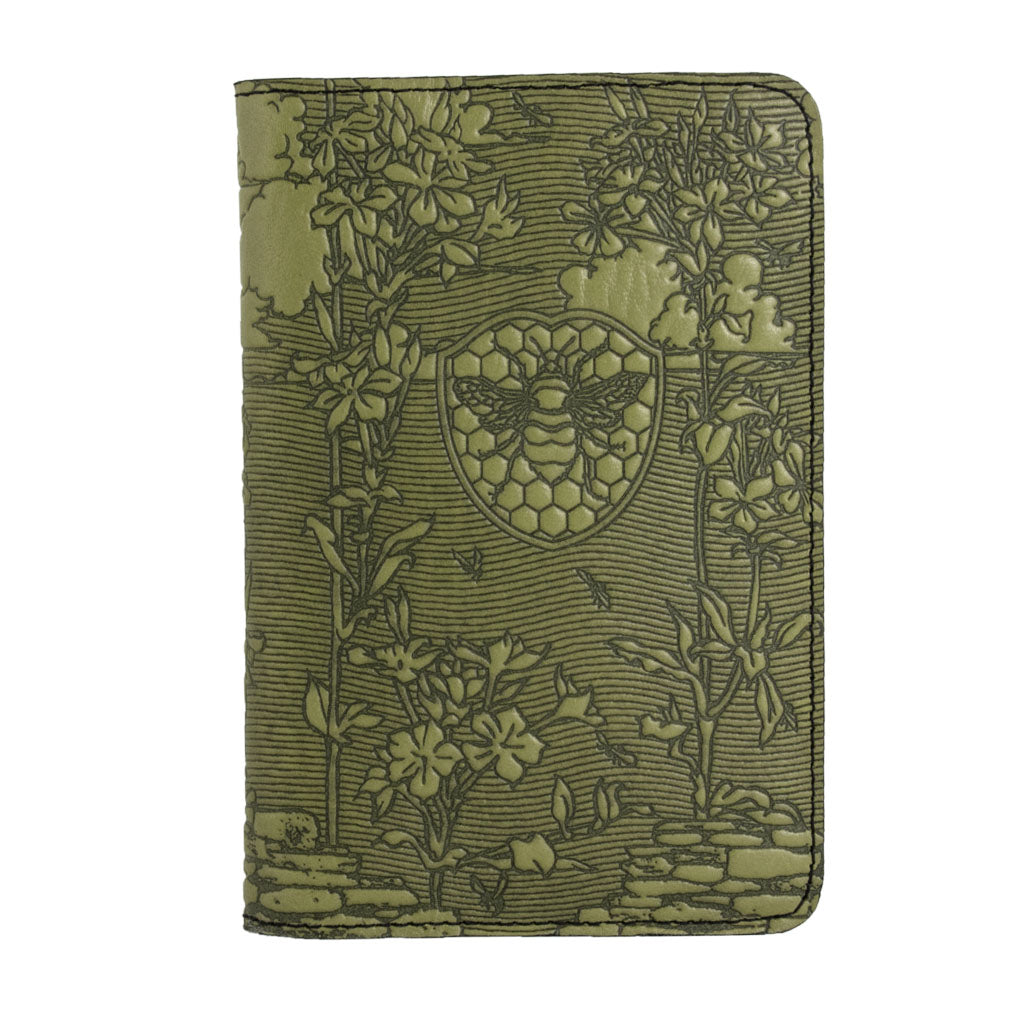The image depicts a rectangular, olive-green leather cover—potentially a diary, wallet, or pouch—featuring intricate designs. The top-right and bottom-right corners of the cover are gracefully curved, and stitching runs around the edges, excluding the left side, which serves as the opening hinge. Central to the design is a shield-like shape adorned with a honeycomb pattern and a bee, flanked by embroidered images of plants with flowers and leaves. Additional floral motifs and plants appear near the bottom, growing atop designs resembling rocks or bricks. The upper part of the cover includes cloud patterns, while the entirety of the cover is accentuated with horizontal black wavy lines, adding depth and texture.